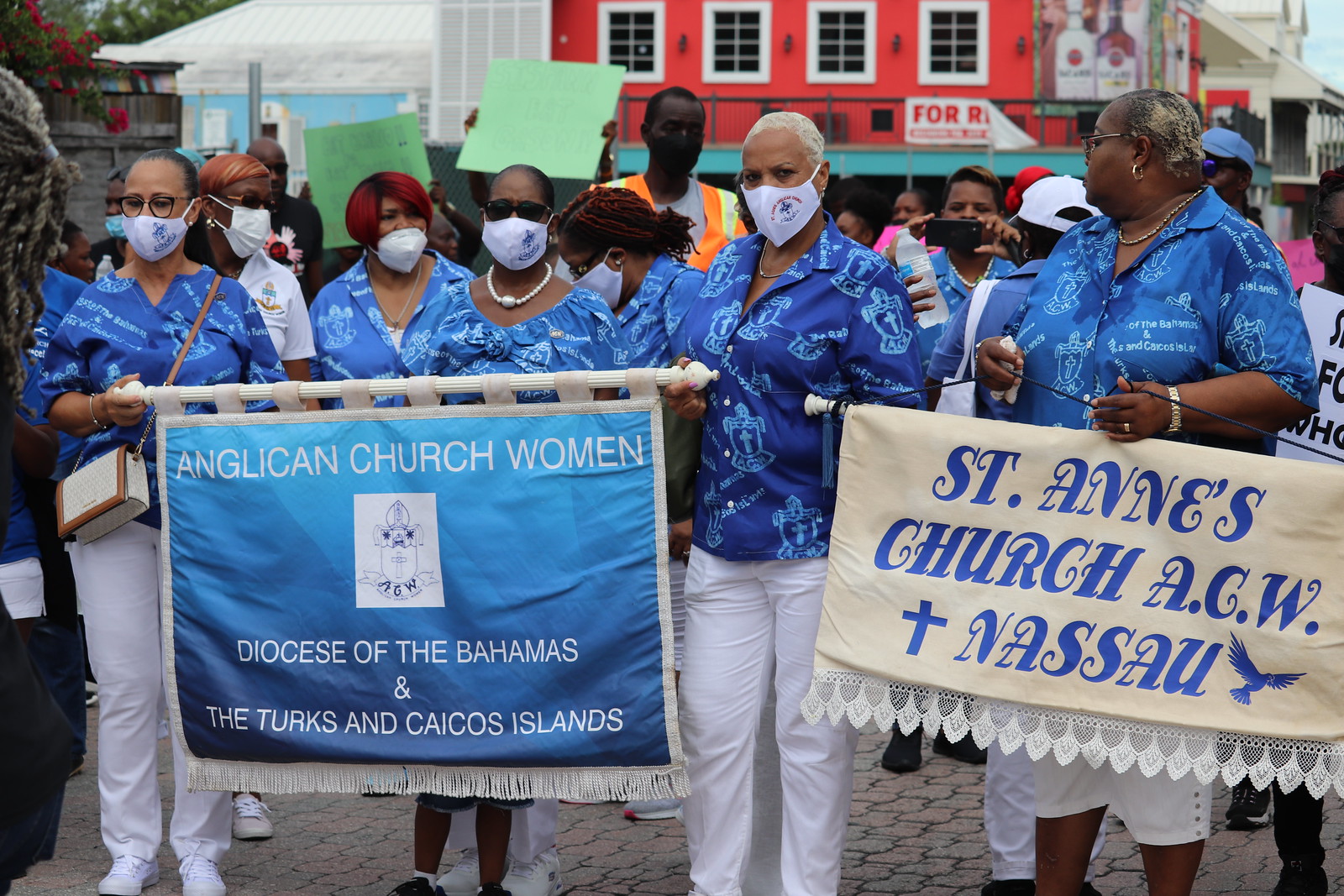In this photo, a group of women, all African American, are gathered outside what appears to be their church, participating in a parade or march. They are standing in a paved street on a slightly cloudy day, in a city setting with a red building featuring white windows and a "for rent" sign in the background. The women are uniformly dressed in blue button-down shirts adorned with crosses and the letters "ACW," symbolizing the Anglican Church Women. Each woman also wears a white COVID mask. At the forefront, they hold two large banners: the one on the left reads "Anglican Church Women, Diocese of the Bahamas and the Turks and Caicos Islands," with blue background and white text, while the one on the right reads "St. Anne's Church ACW Nassau." This banner is white with blue text and includes a cross and a flying bird. A tall man is visible in the background, contributing to the diverse and communal atmosphere.